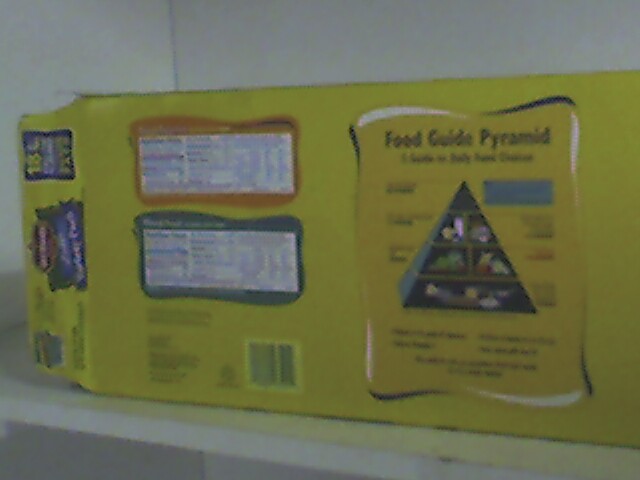This image features a brightly colored food guide pyramid, designed as an infographic to illustrate daily dietary recommendations. The pyramid showcases a variety of food groups, though the exact items are indistinguishable. The background of the box is yellow, with several blocks of text and labels in different colors. Notably, there is an orange label and a green label, presumably detailing the nutritional information for the contents. 

A barcode is present alongside some minor labeling details. At the top of the box, a colorful label predominantly featuring purple colors can be seen, accompanied by a blue stamp section displaying the number 18. This might indicate a box top, which suggests this packaging is aimed at children or intended for a school lunch program to promote nutrition.